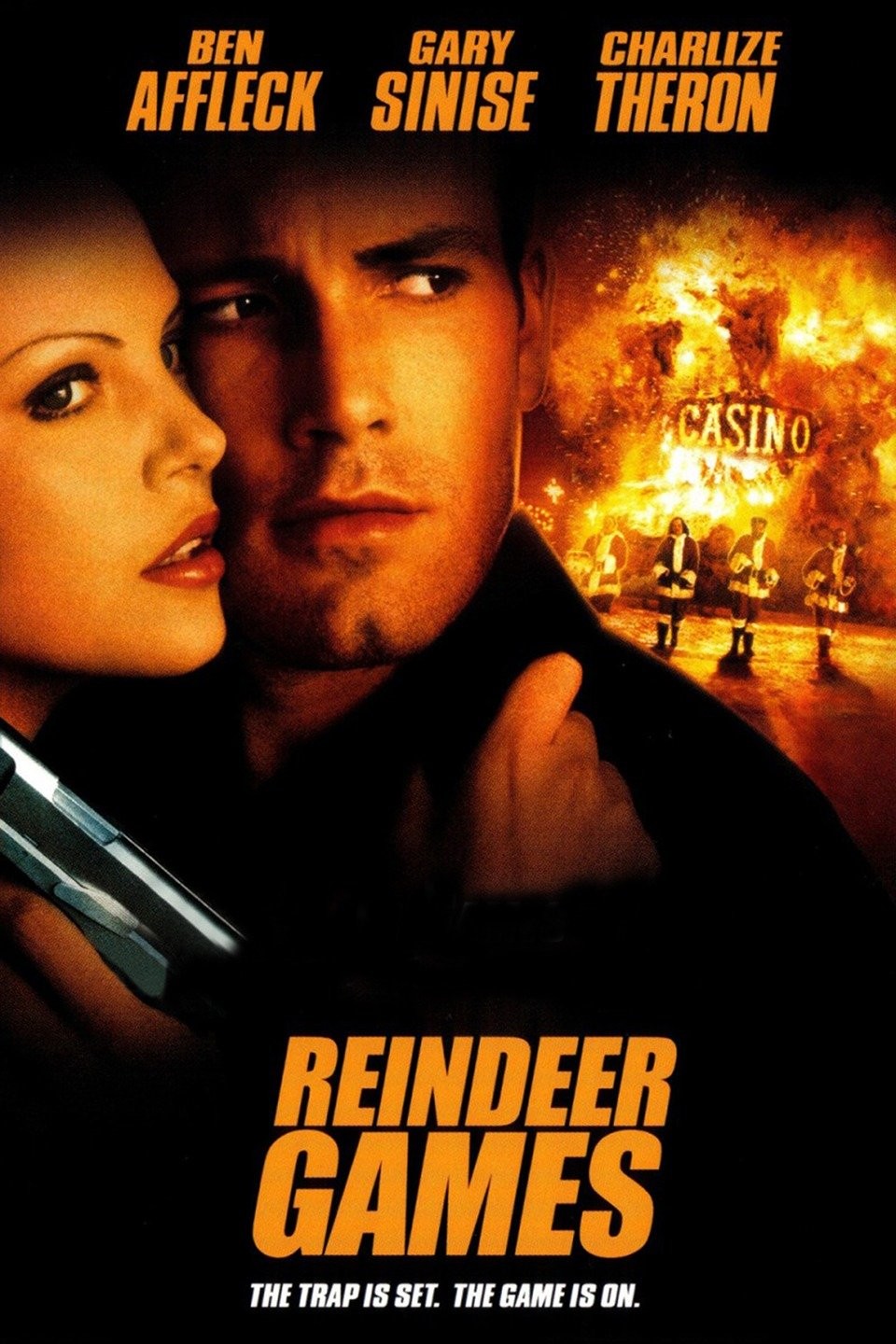The image depicts a detailed and vibrant movie poster for "Reindeer Games," a film featuring stars Ben Affleck, Gary Sinise, and Charlize Theron. Dominating the top section of the poster, their names are prominently displayed in an orange color. Below the names, a photograph captures a close-up of Ben Affleck and Charlize Theron on the left side, appearing intimate with their faces close together. To the right of them, a dramatic scene unfolds showing a burning casino with the text "Casino" visible amidst the flames. In front of this chaos, four people are dressed in Santa Claus suits, adding an intriguing element to the visual narrative. The bottom of the poster displays the movie's title, "Reindeer Games," in bold orange letters, with the tagline "The trap is set, the game is on" clearly visible in white beneath the title. The poster's color palette includes shades of beige, tan, gray, orangish-yellow, white, yellow, and red, all contributing to a dramatic and visually engaging composition.